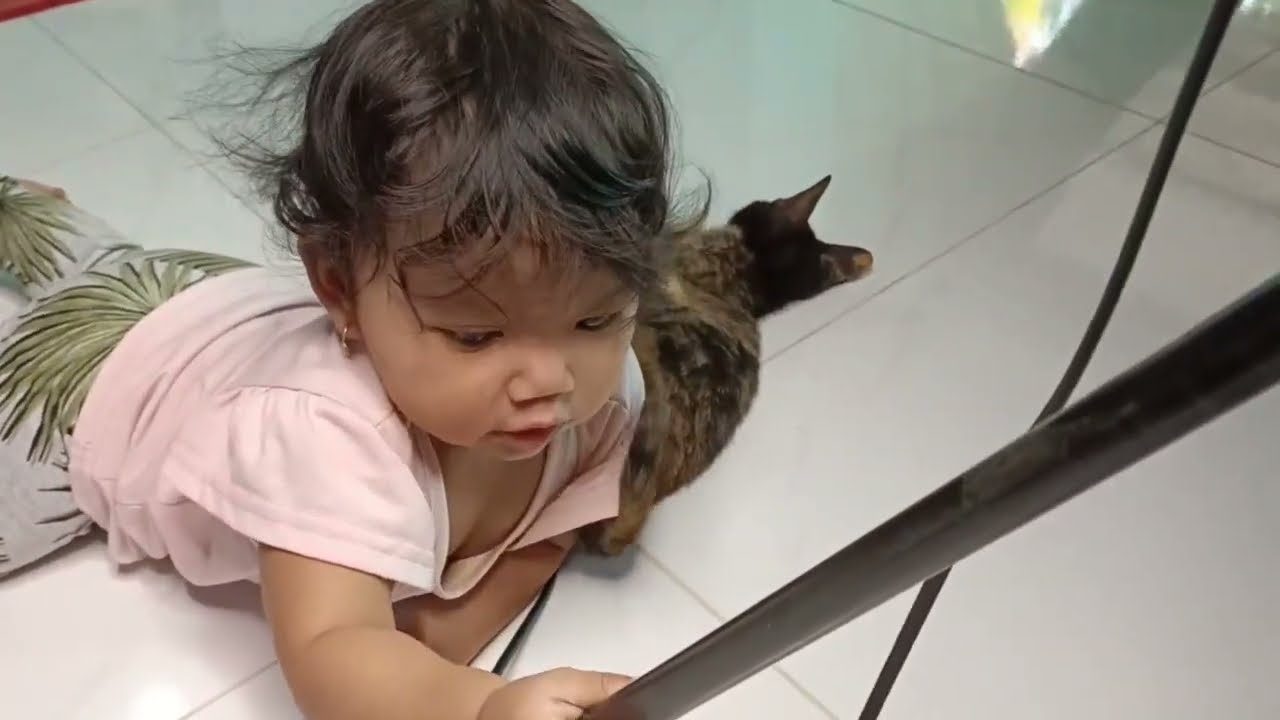In an indoor setting, a very young toddler with dark, slightly messy brown hair adorned with a small gold hoop earring is lying on their stomach on a white tiled floor. The child, likely of Asian descent, wears a light pink shirt and pants decorated with green palm leaf patterns. Their left hand grips a pole or rod extending diagonally from the bottom center to the middle right of the image, with a black cord visible in the frame. Positioned centrally behind the child is a mottled brown, black, and gray cat, its black head featuring beige-tipped ears. The cat lounges sideways on the tile floor, seemingly gazing towards the outside, as indicated by the faint reflection visible in the tile. In the upper left corner of the image, a hint of red can be seen. The toddler, meanwhile, appears to be pointing towards the cat, facing the camera and creating a charming and intimate moment captured in this cozy indoor scene.